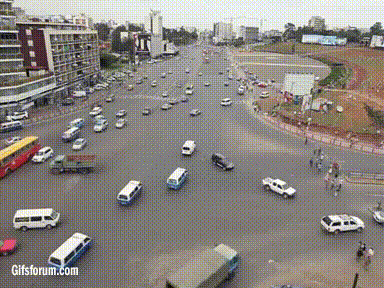An overhead view captures a sprawling network of large, wide roads converging chaotically without any visible road markings or traffic signals. The scene is a whirl of activity with numerous vehicles moving in all directions—some going straight, others turning right or left—creating a sense of utter disarray. Amid this vehicular mayhem, a significant number of cars and trucks navigate the roads, while pedestrians nonchalantly stroll across, adding to the perilous environment. In the upper left corner of the image, a row of buildings borders the road, offering a semblance of order. The roads are teeming with not just personal cars but a variety of larger vehicles, including buses and trucks, indicating heavy traffic volume and diverse transportation modes. The absence of any form of traffic control transforms the scene into a snapshot of chaotic urban motion.